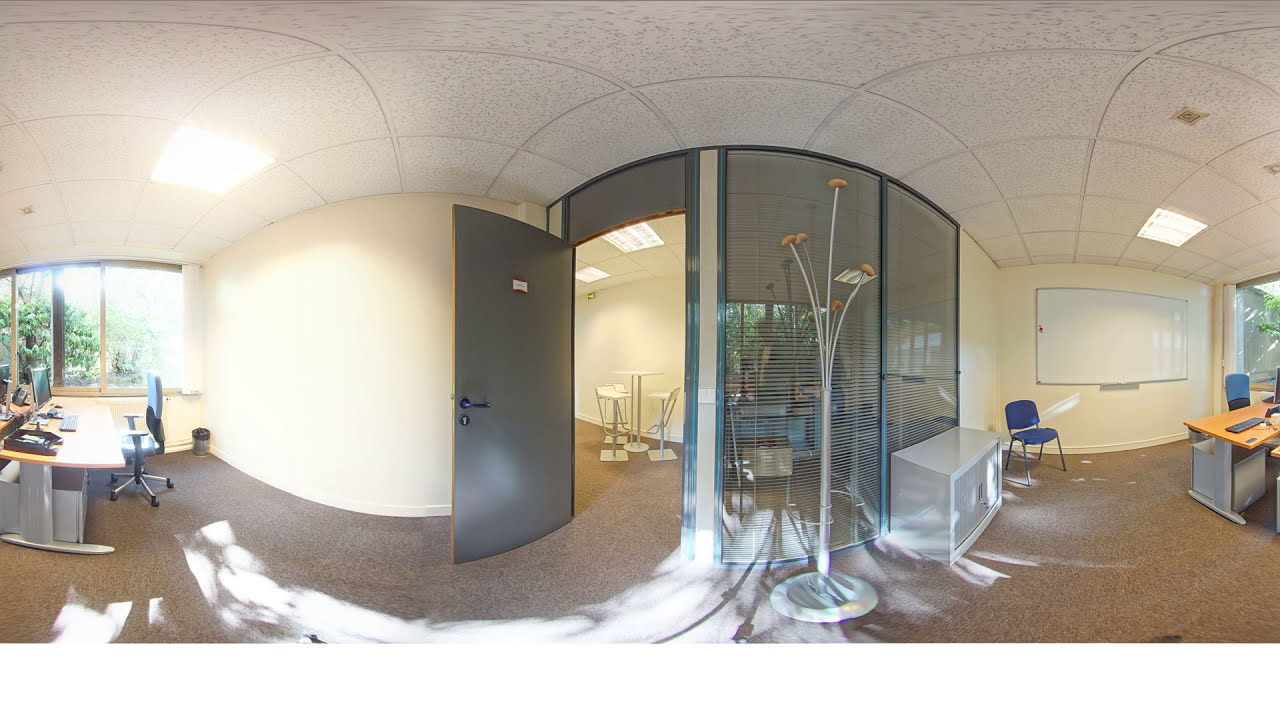This image depicts a modern business office with an open floor plan. The room is horizontally rectangular, featuring light gray ceilings adorned with square lights. The walls are painted a light tan color. On the left-hand side, a large window illuminates a light tan business desk positioned in front of it, with a blue office chair and laptops on the desk. The floor is covered in medium-dark brown, flat carpet. Central to the room is a doorway with a large dark gray door, which opens into a smaller office space furnished with a small white table and pedestal chairs. The doorway is flanked by glass parts of a wall with blinds. Adjacent to the entrance of the smaller office, there's a tall, metal sculpture resembling a coat rack, branching out like a tree. To the right, another business desk, accompanied by blue chairs, sits in front of a large whiteboard mounted on the wall. Sunlight pours in through the left window, casting rays that create a pattern on the carpet. The overall ambiance of the room is bright and functional, with an efficient layout and modern furnishings.